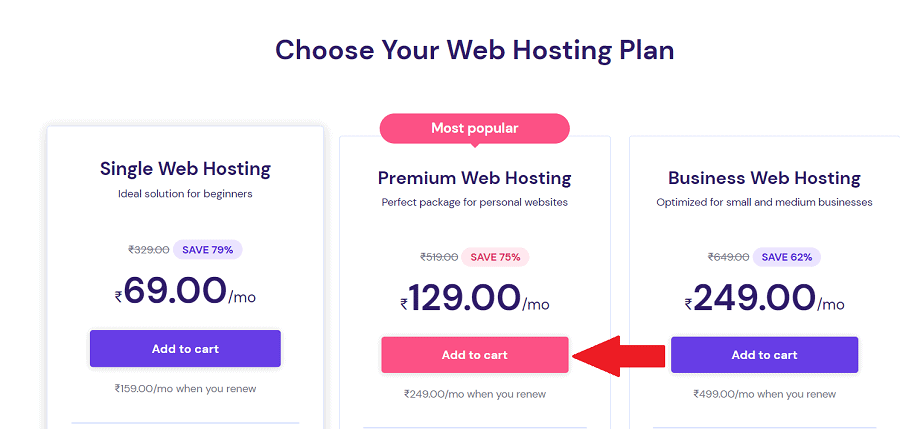The image displays a web hosting plan selection page with three tiers of service offerings, each tailored to different needs and accompanied by a savings percentage. The tiers are listed from left to right, each with distinct colors for their 'Add to Cart' buttons.

1. **Single Web Hosting**: Ideal for beginners, this plan promises a significant savings of 79%. The current price is 69.00 (currency unknown) per month, with the 'Add to Cart' button depicted in blue.

2. **Premium Web Hosting**: Labeled as the most popular choice, this package is designed for personal websites. It offers a 75% discount, bringing the price to 129.00 (currency unknown) per month. The 'Add to Cart' button for this tier is highlighted in pink. Additionally, a red arrow emphasizes this middle option, directing attention towards the pink button.

3. **Business Web Hosting**: Optimized for small to medium businesses, this tier costs 249.00 (currency unknown) per month. Like the Single Web Hosting plan, the 'Add to Cart' button is blue.

The overarching implication is for users to select a plan that aligns with their website needs and expected user traffic, with a specific visual emphasis on the most popular, middle-tiered Premium Web Hosting plan.